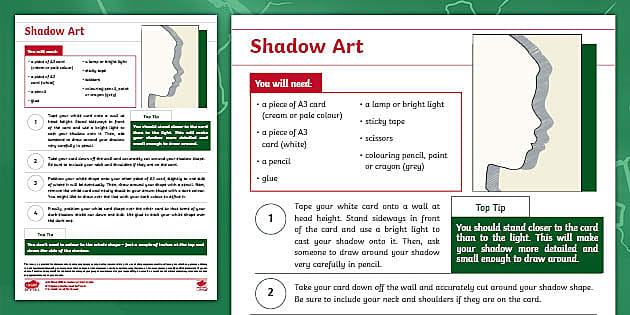The image depicts a detailed presentation on how to create shadow art, emphasizing a comprehensive set of instructions. The entire piece is horizontally rectangular, featuring a green background and border. On the left side, there is a vertically rectangular section containing the step-by-step guide, while on the right side, there is a square section showcasing the final shadow art product. Both sections are labeled "shadow art."

The instructions start with a list of required materials including a piece of A3 card in white or cream color, a pencil, glue, a lamp or bright light, sticky tape, scissors, and coloring tools like paint or crayons in gray. The first step involves taping the white card onto a wall at head height and standing sideways in front of it to cast a shadow with the bright light. Someone else will then carefully trace around the shadow. A top tip suggests standing closer to the card than to the light for a more detailed and manageable shadow.

The second step instructs to take the card down and accurately cut around the traced shadow, ensuring the neck and shoulders are included if they were part of the silhouette. The right section of the image displays the resulting shadow art with a silhouette of a child's profile in white, outlined in black with an accompanying shadow, demonstrating the final effect.